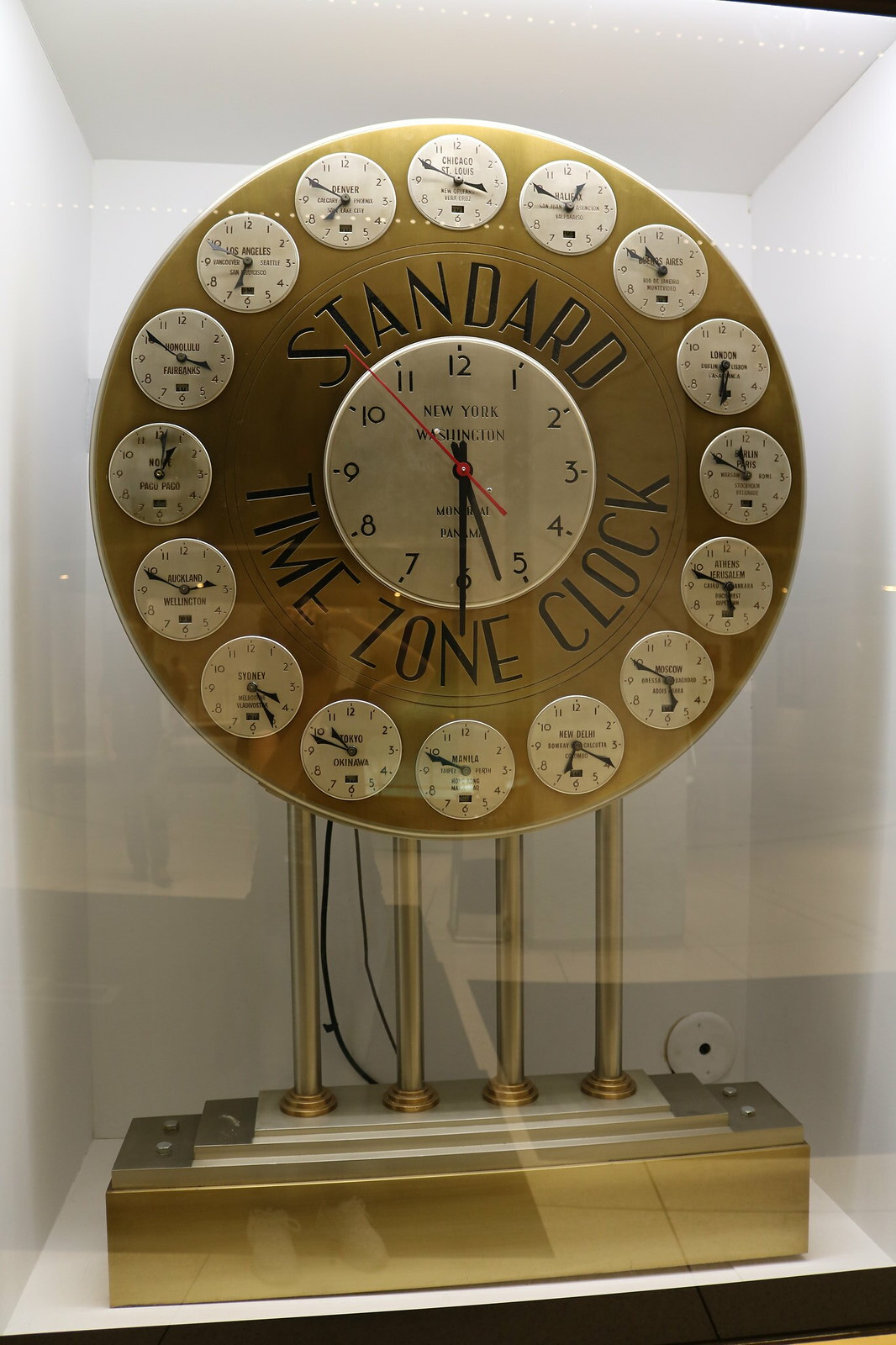The image features an elegant gold clock encased behind a layer of protective plexiglass, evident from the reflections of the surrounding environment visible on the glass. The clock is set within a display case with pristine white sides and a polished brown exterior. The centerpiece of the display is a striking timepiece that prominently displays the current New York time at 5:30, with a distinctive red second hand and black hour and minute hands. Etched into the golden frame surrounding the main clock face is the inscription "Standard Time Zone Clock." Encircling this central clock are several smaller clocks, each representing different global time zones. The entire arrangement is mounted on a set of four brass supports that elevate it above a long, elegant brass box, adding to its sophisticated presentation.